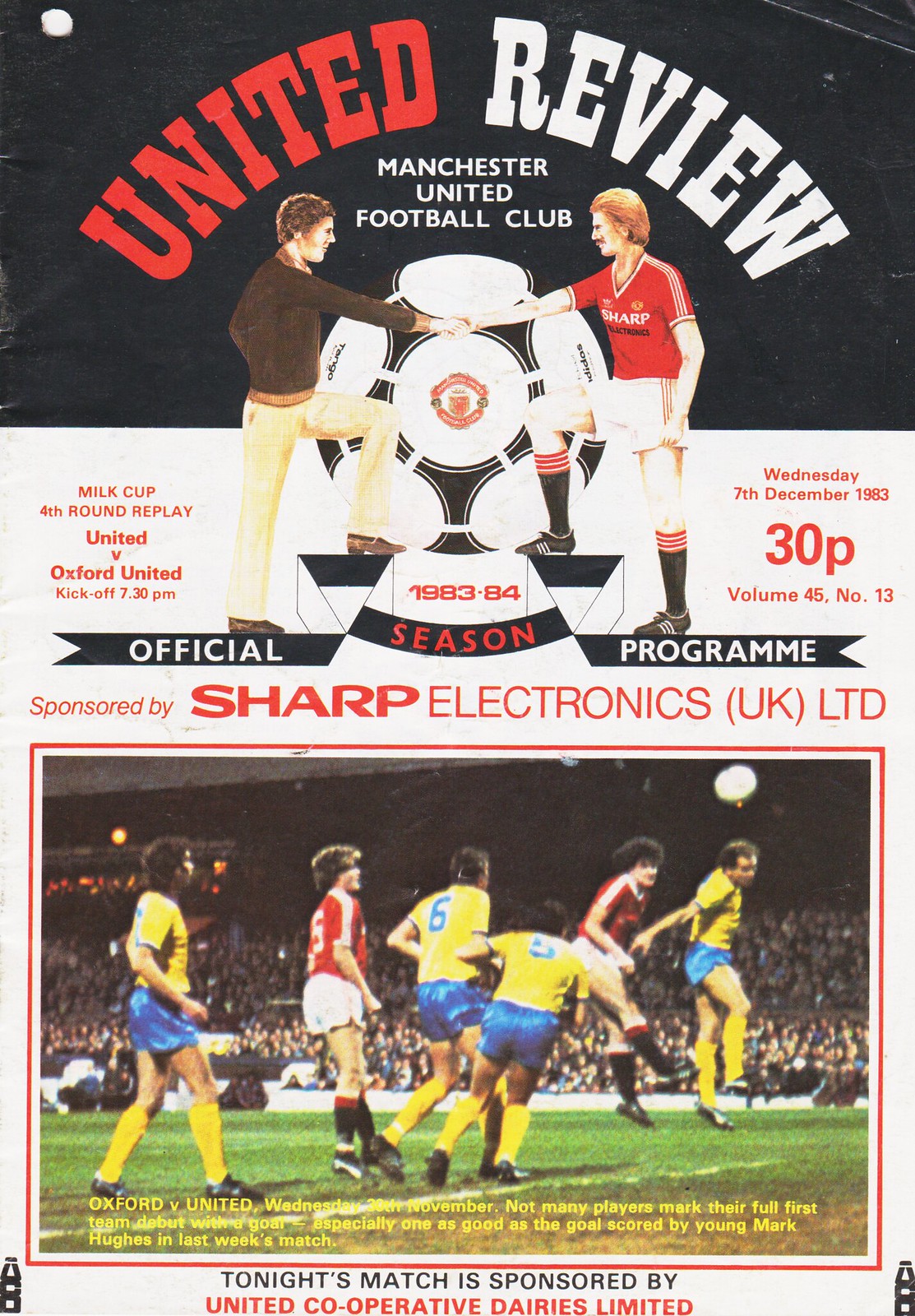This is a detailed front cover of an official sport program for a Manchester United Football Club match. At the top, in bold white text on a black header, it states "United Review, Manchester United Football Club." Beneath this header, the program announces in red lettering over a white background: "Milk Cup Fourth Round Replay: United versus Oxford United," and lists the date as "Wednesday, 7th December 1983" with the price "30p". The middle section prominently features an image capturing two teams during a match; one team is in yellow and blue uniforms, and the other team is in red and white. The players, including one heading a white soccer ball, are set against a backdrop of a packed stadium. At the bottom, the text mentions that "Tonight's match is sponsored by Sharp Electronic UK Ltd and United Cooperative Dairies Ltd". The phrases "Official Program" are recurring in red and white throughout the design, emphasizing its formal nature.